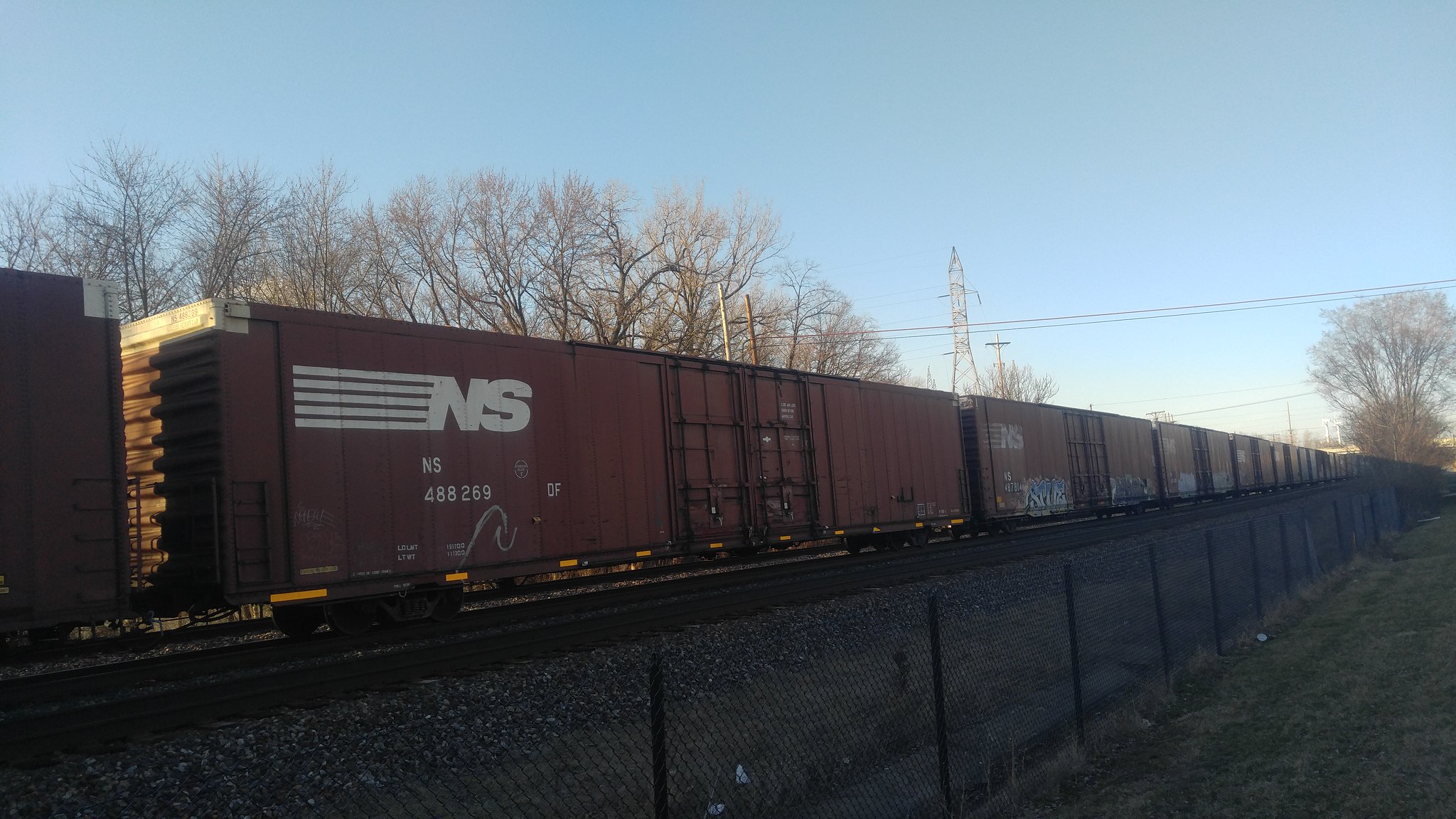In this detailed photograph, we see a lengthy freight train on black train tracks that extend from the left side of the image towards a vanishing point on the right. The train cars are uniformly dark red with a white logo featuring the letters "NS" and white identification numbers, such as 488269, adorning their sides. While the closest cars have minimal graffiti, some show signs of it. Behind the train, tall, leafless trees stretch upwards, indicating a dormant season. The sky overhead is a vibrant, clear blue, transitioning to a lighter hue near the horizon, suggesting early morning or afternoon light.

The lower right corner of the image shows a green but dark grass lawn, bordered by a black chain-link fence that stands about chest-high. Some white debris is stuck in the fence's holes. Beyond the fence, there's a mixture of plant life and pebbles leading to the tracks. The overall composition captures the expansive, serene, and somewhat industrial landscape with remarkable clarity and depth.